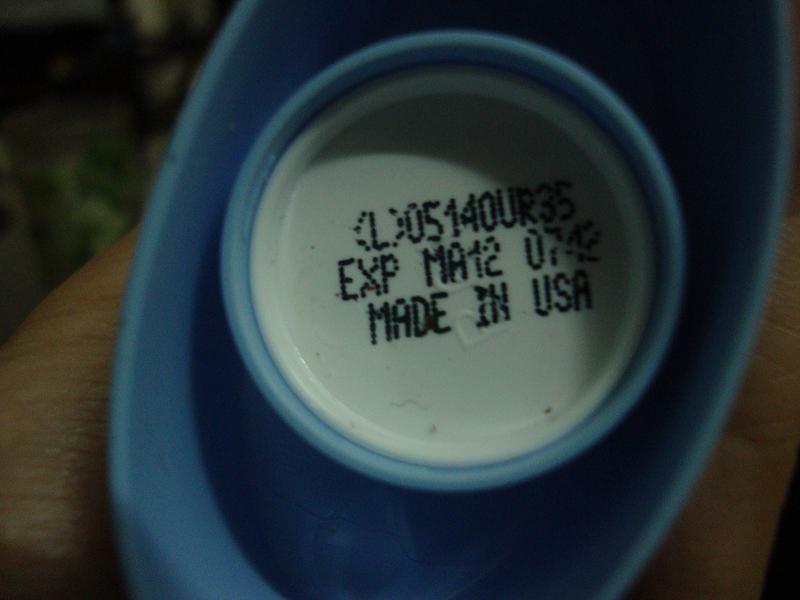The image depicts a close-up of the bottom of a light blue deodorant container. The container is held in a small blue plastic dish resembling a soap dish, possibly by someone's hand, partially visible in the frame. Centered in the bottom of the deodorant container is a white circular area featuring black printed text, including a serial number, an expiry date labeled "MA 12," the number "0742," and the words "Made in USA." The setup is placed on a flat wooden surface that could be a table or chopping block. The overall scene focuses on the detailed markings at the base of the deodorant, highlighting the circular design and the contrast between the blue and white elements.